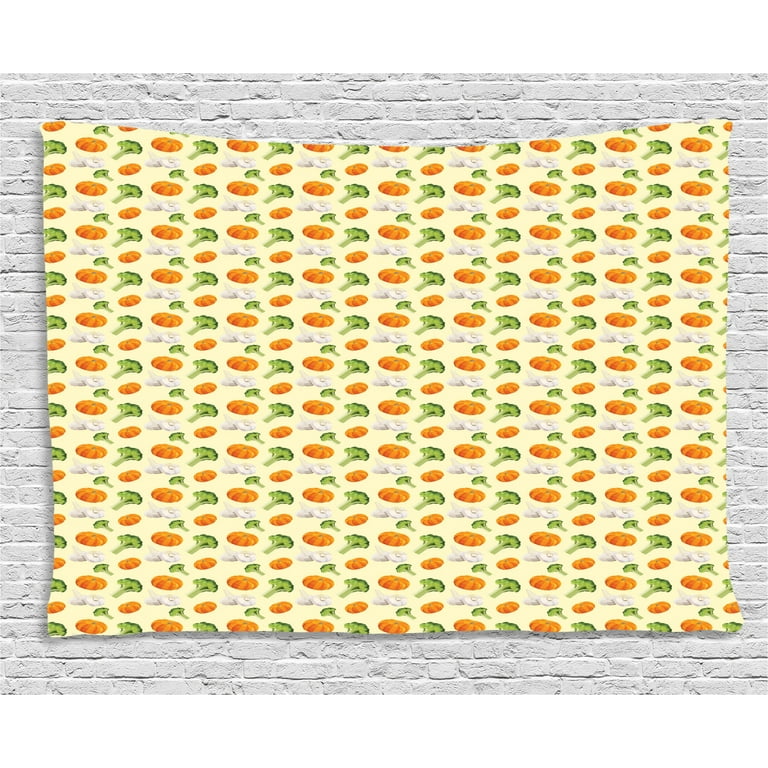The image depicts a large piece of fabric hanging on a white brick wall, adorned with an intricate, computer-generated pattern. The design features a repetitive and alternating series of vegetables: pumpkins, broccoli, and cauliflower or possibly garlic bulbs. The pumpkins are orange with green stems, the broccoli is green with darker florets, and the garlic or cauliflower is a beige-white hue. These vegetables are depicted in a 2D style with shading to provide a semblance of depth. The pattern is arranged in horizontal rows with minimal spacing, and variations include smaller versions of the pumpkins and broccoli. The entire pattern is set against a yellowish-beige background, creating a striking visual contrast against the textured brick wall.